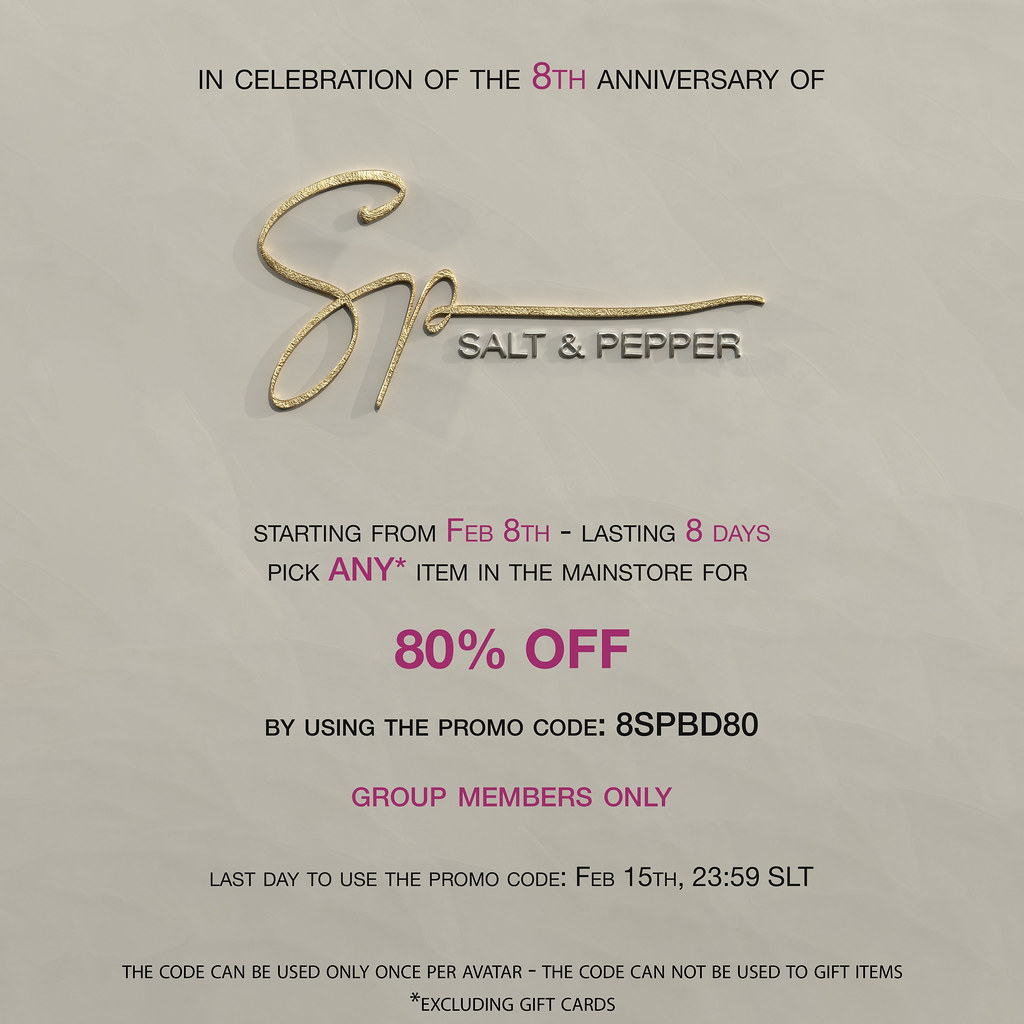The image is a promotional card celebrating the 8th anniversary of the brand Salt and Pepper. It has a square layout with a light gray to beige background. The top of the card reads "In celebration of the 8th anniversary of" in black text, with the word "eighth" highlighted in purple. Below this header is a large gold insignia featuring the letters "SP," with a silver or gray text "Salt and Pepper" written beneath it. 

The promotion details are positioned under the brand name, with varying colored text to emphasize key points. In black and purple, it announces: "Starting from February 8th, lasting eight days, pick any item in the main store for 80% off by using the promo code 8SPBD80." Critical details such as "February 8th," "eight days," and "80% off" are highlighted in purple. A note follows stating, "Group members only," also in purple. 

A disclaimer at the card's bottom, in small black print, specifies: "The code can be used only once per avatar, cannot be used to gift items, and excludes gift cards." The final detail mentions the promo code's expiration: "Last day to use the promo code is February 15th, 23:59 SLT," with "SLT" possibly referring to Salt Lake Time.